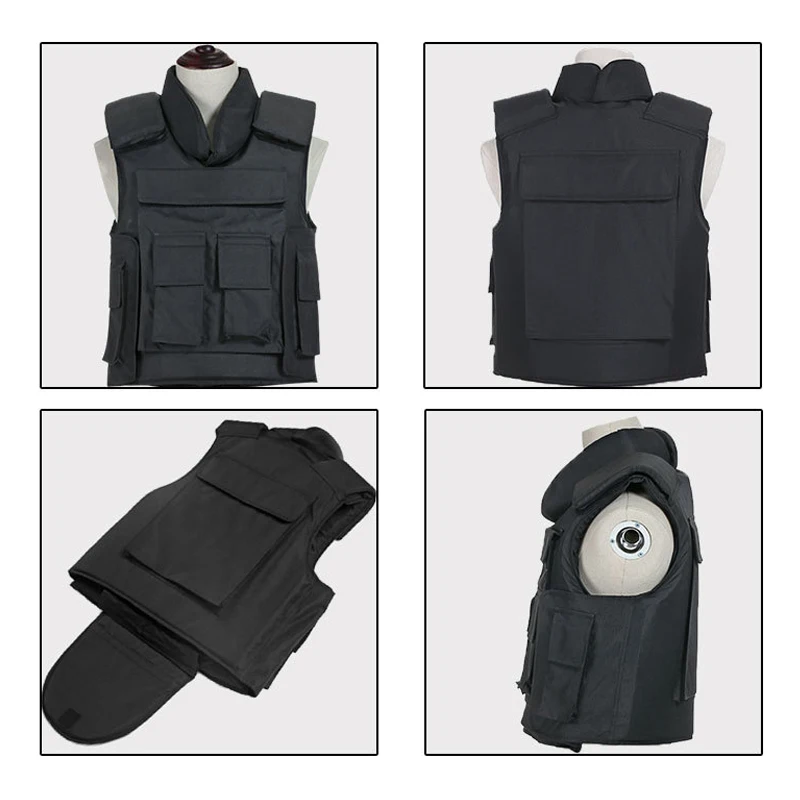This composite image displays a detailed view of a black tactical bulletproof vest from four different angles, each illustrating distinct features of the vest. The top left quadrant shows the front view of the vest on a white mannequin, highlighting large padded shoulder straps and a padded neck collar. The front is equipped with four smaller pouches and a large central pouch. The top right quadrant provides the back view of the vest, again on the mannequin, revealing a large back pocket and the extensive padding around the shoulders and neck area. The bottom left quadrant showcases the vest laid flat, exposing an open flap with Velcro closure at the bottom and emphasizing its versatility and storage capabilities. Finally, the bottom right quadrant presents a side view on the mannequin, offering a comprehensive look at the vest's structure, including the side pouches and overall fit. The entire setup is against a grayish-white background, enhancing the visibility of the vest's all-black design, which appears robust, heavily padded, and potentially made from Kevlar or a similar bulletproof material.